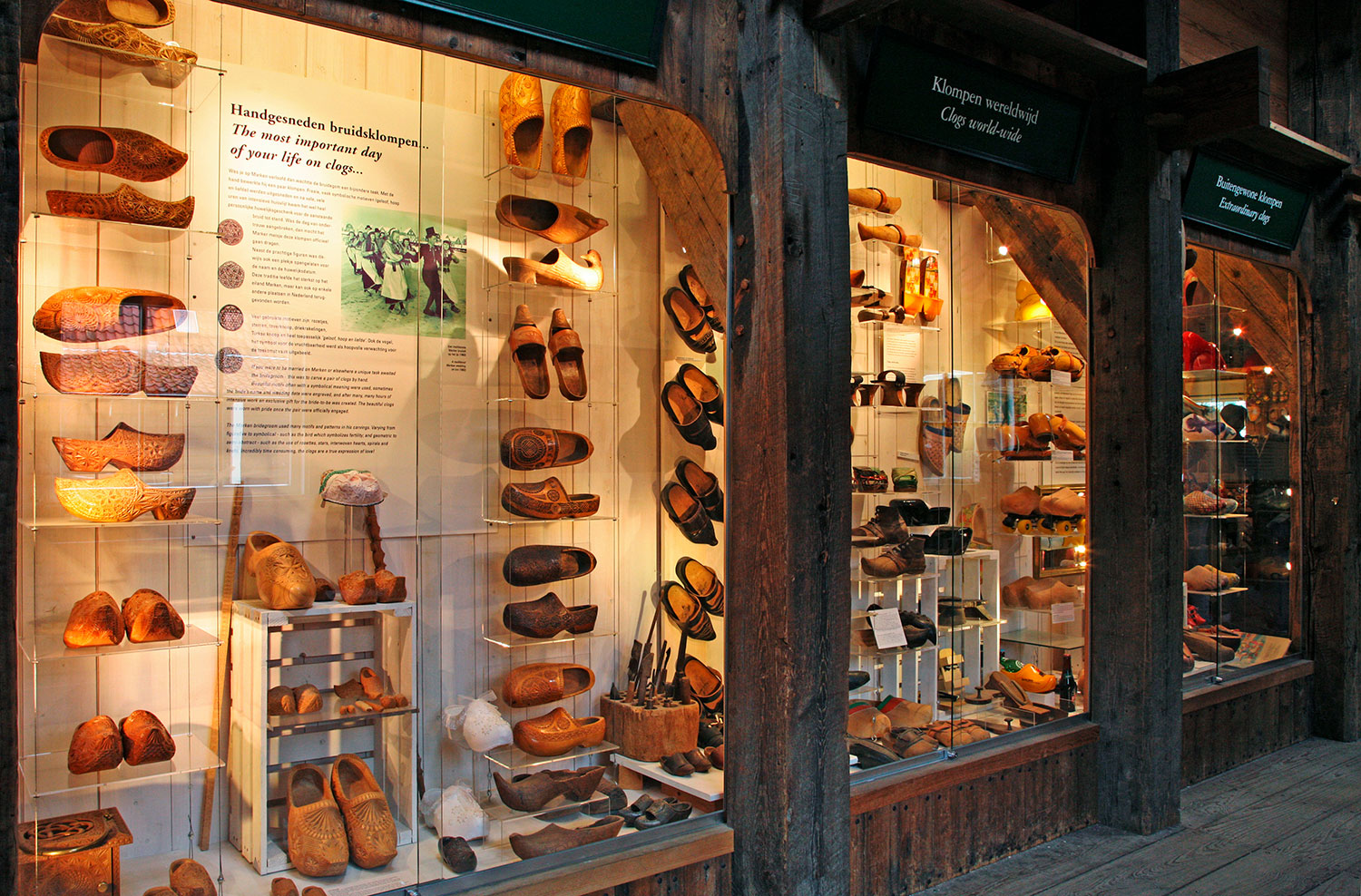This image captures a detailed display, likely part of a shoe museum or a specialized shoe store, showcasing intricately crafted clogs. The exhibition is divided into three distinct sections, each enclosed in large glass cases framed by a dark, thick wooden trim. The gray, brick pavement beneath adds to the sophisticated ambiance.

Within these glass cases, several pairs of clogs are prominently arranged on clear, plastic platforms and shelves, highlighting their craftsmanship. Each section features text above and below the display. Notably, one section is titled "Clogs Worldwide," and another reads "Extraordinary Clogs," though the text in the third section is not legible.

Accompanying the shoes in the first case is an inscription, "The Most Important Day of Your Life on Clogs," alongside an old black-and-white photograph of a man and woman, seemingly in the midst of a dance. The history and origin of the shoes are detailed, likely giving insights into their cultural significance and manufacturing background. The clogs, primarily made of brown wood with some having black exteriors, are showcased as well-crafted pieces, offering a glimpse into the traditional art of clog making.